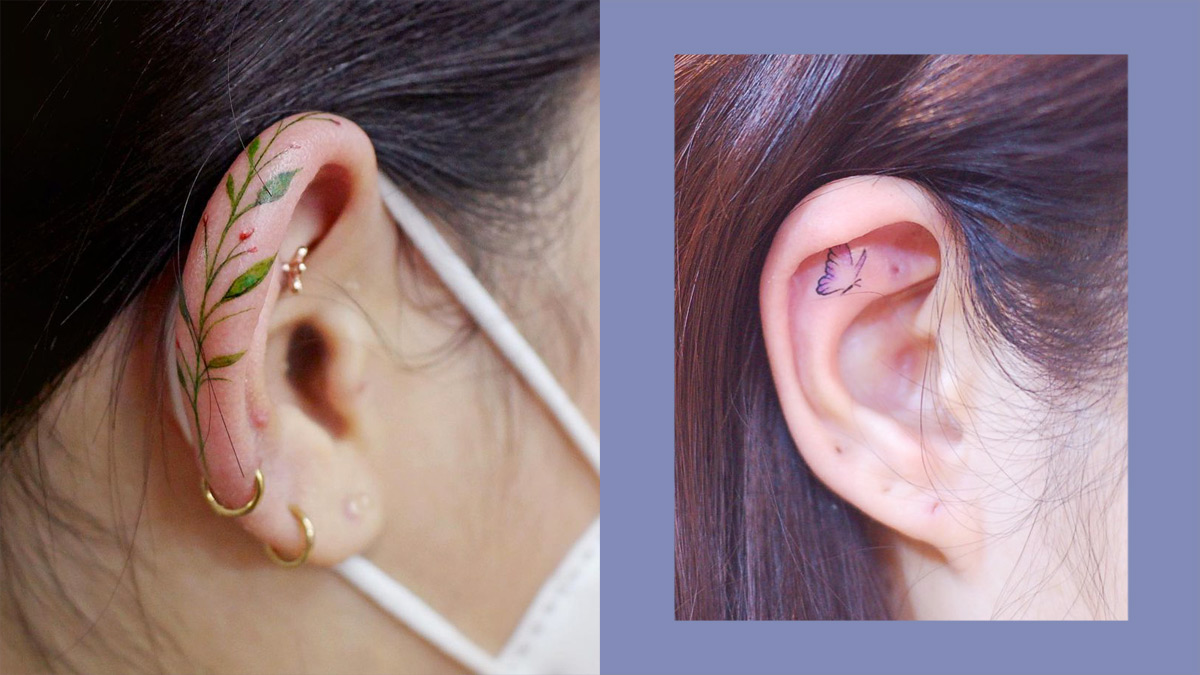The image depicts two side-by-side close-up photos of women’s ears adorned with tattoos and piercings. The left image features an ear with black hair pulled back, revealing a white mask strap looped around it. The ear sports a tattoo of a green plant with red flowers along the rim and is adorned with two gold ring piercings in the earlobe. In contrast, the right image shows an ear with medium brown hair, displaying piercing holes but no earrings. This ear has a delicate outline of a purple butterfly tattooed inside. Both images highlight the intricacy and decorative nature of the ear tattoos, possibly temporary, against the backdrop of different hair colors and piercings.